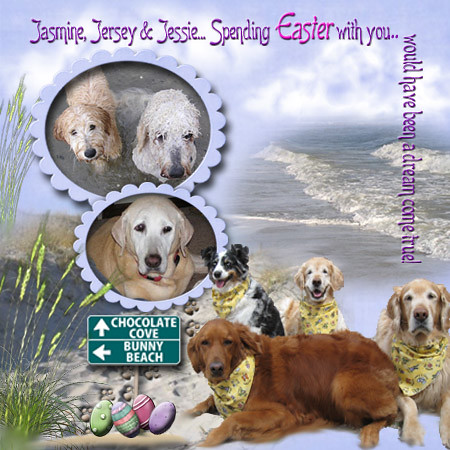This image captures an intricately designed Easter greeting card featuring adorable dog photos. Dominating the top, pink and purple text reads: "Jasmine, Jersey, and Jesse spending Easter with you... would have been a dream come true!" This heartfelt message is accompanied by a collage of various dogs, including golden retrievers and other breeds, against a backdrop that combines real-life and cartoon elements. Notable details include a whimsical green sign pointing to "Chocolate Cove" and "Bunny Beach," framed by scenic images of sand, Easter eggs, flowers, and grass growing on a beach. The overall design is both playful and nostalgic, seamlessly blending images of Jasmine, Jersey, and Jesse with stock photos of four additional dogs. The card even features a real map, further enhancing its charm and uniqueness.